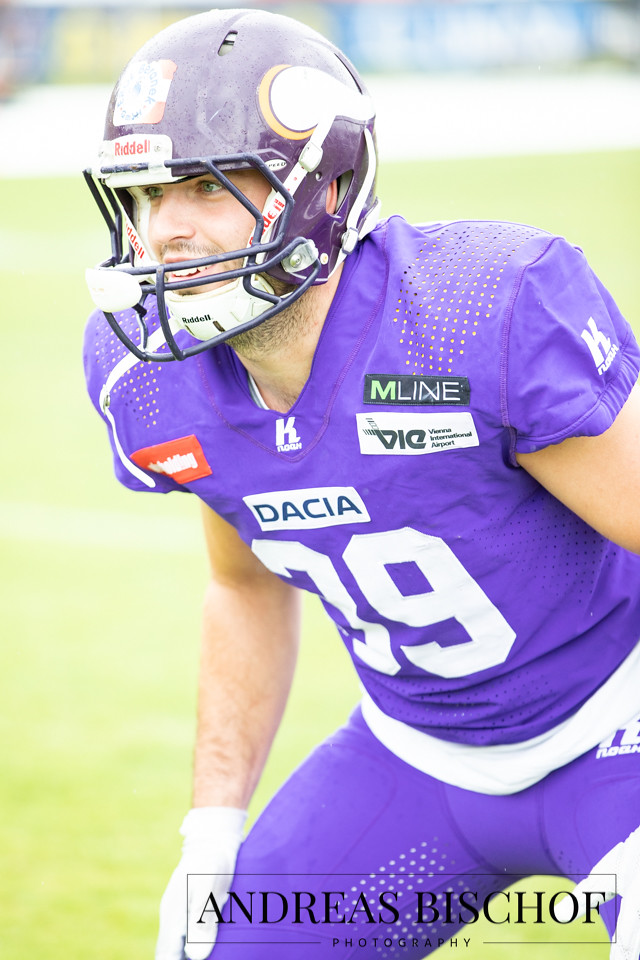The photograph captures a young Caucasian man, a football player for the Dacia Vienna Vikings, dressed in a vibrant purple uniform with white lettering and a maroon Riddell helmet. His uniform is emblazoned with various sponsor logos, including those for Dacia, M-LINE, and Vienna International Airport. The player's clean uniform and the setting—a green, out-of-focus football field background—suggest that this is a posed shot rather than an action shot during a game. The player, wearing number 39, is squatting as if ready for a play, smiling slightly with visible light eyes and a five o'clock shadow. The bottom of the photo features the watermark "Andreas Bischoff Photography," attributing the image to its photographer.